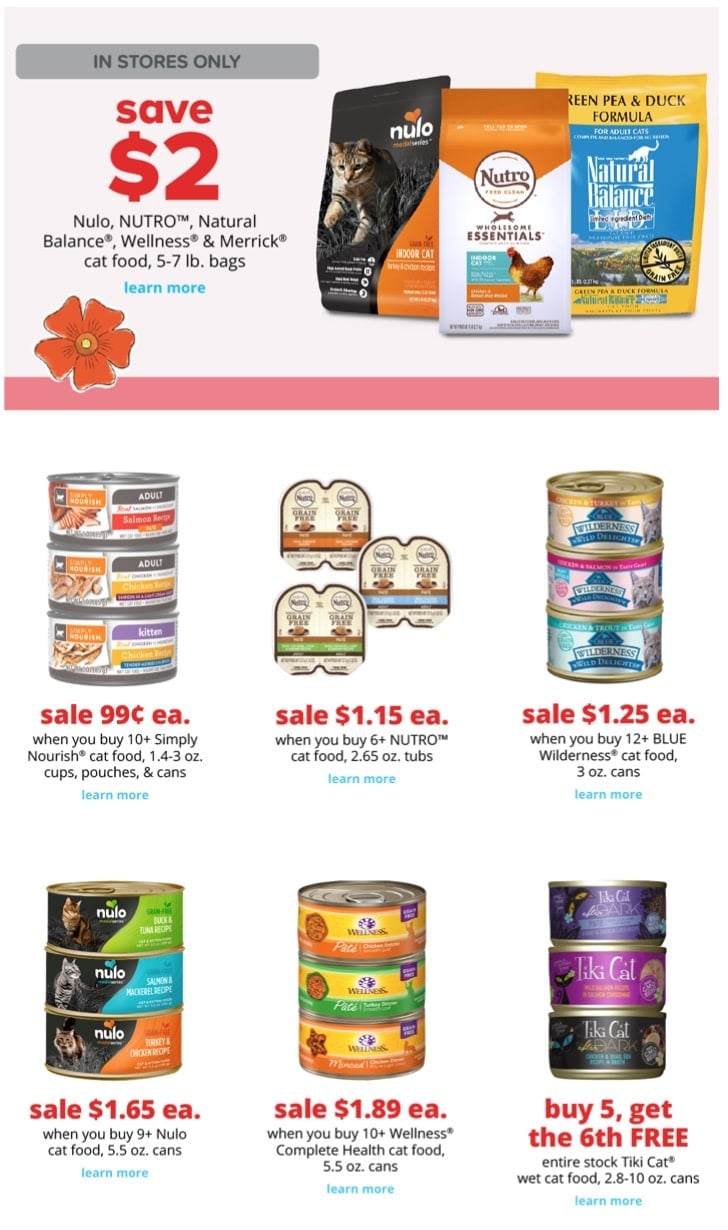This image appears to be an advertisement for pet products, specifically cat food, with multiple offers and promotional deals. 

At the top of the image, there is a gray box with the text "IN STORES ONLY." Beneath this, the advertisement highlights a $2 savings on various brands and types of cat food, specifically "NEW LOW," "Neutral," "Natural Balance," "Wellness," and "Merrick" cat foods, available in 5 to 7-pound bags. A clickable button labeled "LEARN MORE" is displayed just below this information.

To the right of the text, three colorful bags of cat food are prominently featured, each corresponding to the advertised brands: "NEW LOW," "Neutral," and "Natural Balance." These bags are adorned with vibrant images of animals, clearly indicating that the products are intended for pets.

Additionally, the lower section of the image organizes sale items into two rows of three products each:

- **First Row:**
  1. "SALE 99¢ EACH when you buy 10+," featuring Simply Nourish cat food in 1.4 to 3-ounce cups, pouches, and cans.
  2. "SALE $1.15 EACH when you buy 6+," showcasing Neutral cat food in 2.65-ounce tubs.
  3. "SALE $1.25 EACH when you buy 12+," highlighting Blue Wilderness cat food in 3-ounce cans.

- **Second Row:**
  1. "SALE $1.65 EACH when you buy 9+," offering NEW LOW cat food in 5.5-ounce cans.
  2. "SALE $1.89 EACH when you buy 10+," featuring Wellness Complete Health cat food in 5.5-ounce cans.
  3. "BUY 5, GET THE 6TH FREE," for the entire stock of Chewy cat wet cat food, available in 2.8 to 10-ounce cans.

Complementing the array of promotions, the image includes a small graphic of an orange daisy flower near the top, adding a touch of bright color to the advertisement.